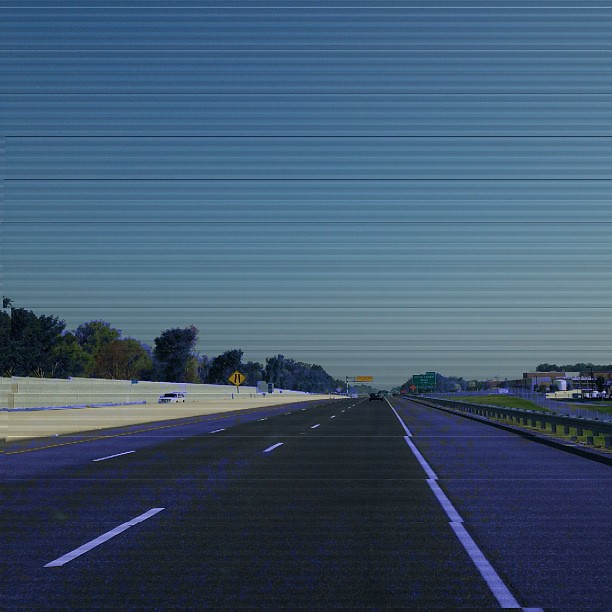This image depicts a bustling interstate scene under a vibrant blue sky. Prominent horizontal gray lines span from the top to the bottom across the entire image, likely indicating the road's lanes and dividers. On the left side, a row of lush trees stands adjacent to a beige-colored barrier lining the edge of the interstate. A white SUV is captured traveling diagonally towards the left side, its front end facing towards the viewer. Nearby, a yellow diamond-shaped sign with two black lines asserts itself on the right of the SUV.

Further to the right of the image, another light beige concrete barrier separates this section of the interstate from a three-lane road. The lanes are neatly divided by white dotted lines, and a thick white border demarcates the shoulder of the road, which is slightly wobbly in appearance. Along the far right of this road, a sturdy guardrail runs parallel to the lanes. In the background, a green exit sign is visible, leading towards some distant buildings surrounded by trees, completing this detailed vista of a typical interstate environment.